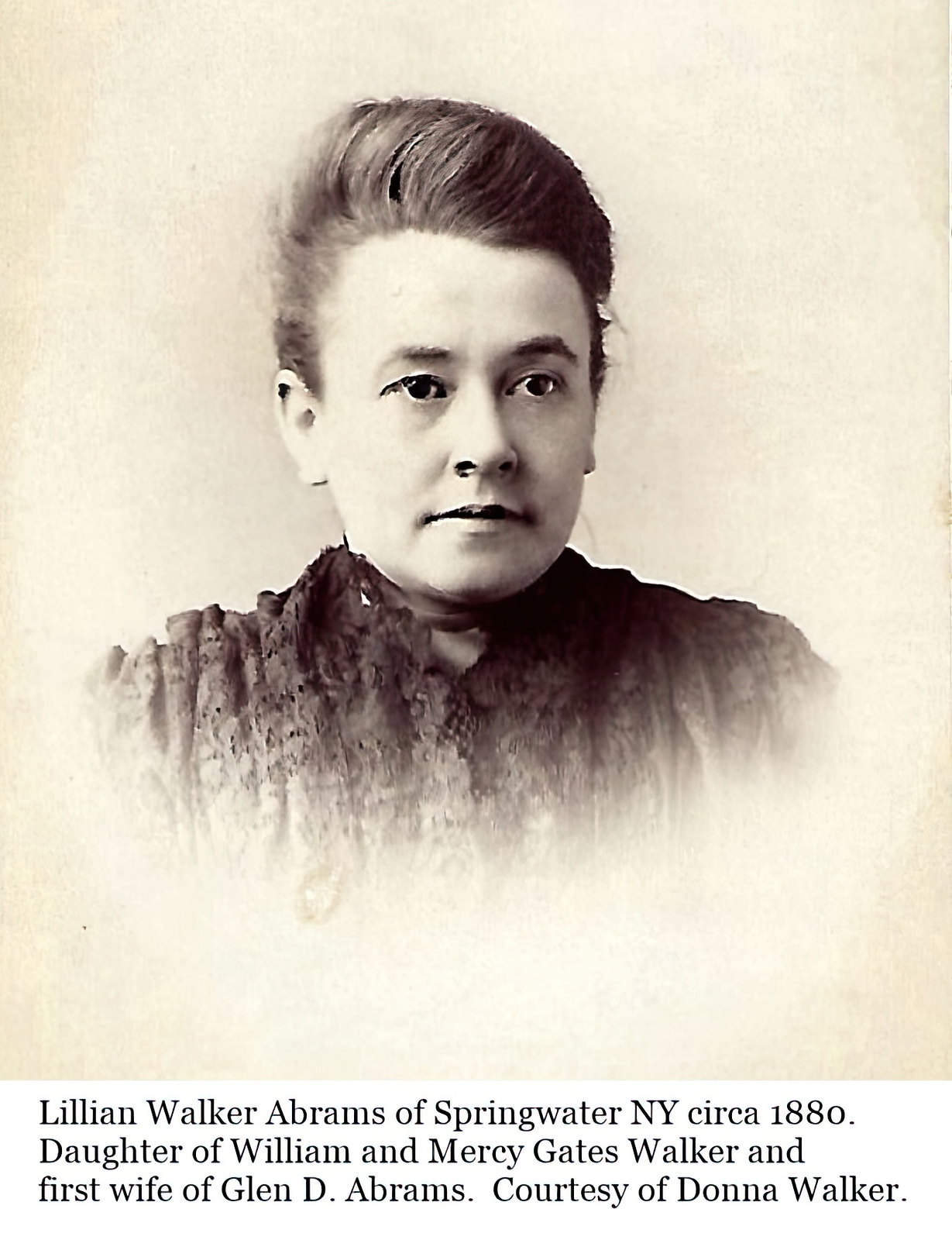This vintage black-and-white photograph, courtesy of Donna Walker, features Lillian Walker Abrams of Springwater, New York, circa 1880. Lillian, the daughter of William and Mercy Gates Walker and the first wife of Glenn D. Abrams, is positioned centrally, showcasing her shoulders and face. She gazes slightly off to the side with her hair stylishly combed up towards the back. Her attire is a very vintage-looking dress with rolling pleats and decorative elements. She dons a distinctive necklace with a ribbon. The background of the photograph presents a neutral, light brown, almost gray tone, setting off the intricate details of her dress and the black-and-white essence of the image.